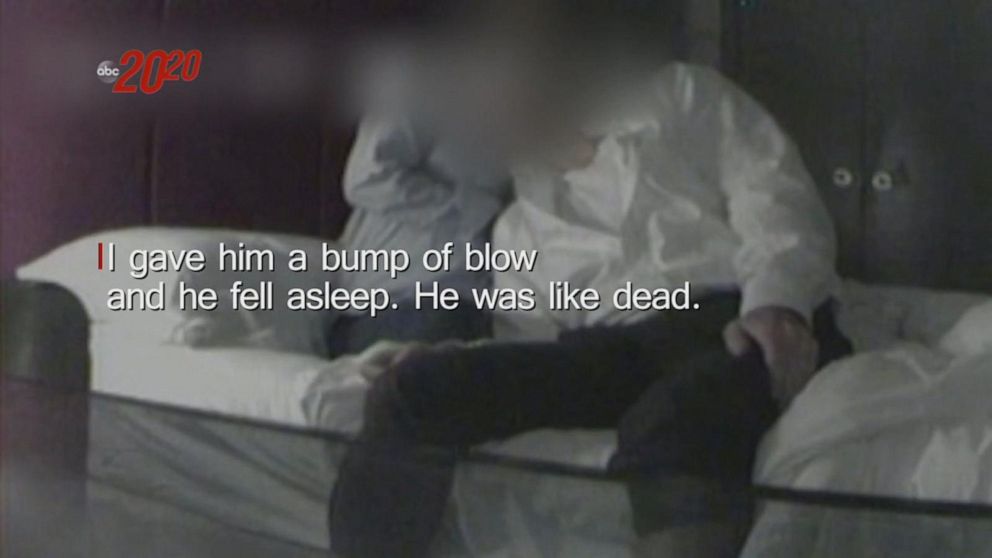The image is a low-quality, blurry screenshot from an ABC 2020 broadcast. Situated in the top left corner of the image is the ABC 2020 logo, with '2020' in red and 'ABC' in black and white. The scene appears to take place in a hotel room with plain white bedding and pillows. In the foreground, a man dressed in a white shirt and black pants sits on the bed, his head blurred out, giving the impression of being either incapacitated or asleep. Next to him on the bed kneels a petite figure, possibly a woman, wearing a blue shirt; her face is also blurred. Behind them, closet doors or a cupboard can be seen. Superimposed across the image is the text, "I gave him a bump of blow and he fell asleep. He was like dead." The image appears to be in black and white, with significant JPEG artifacts, adding to its overall low resolution.